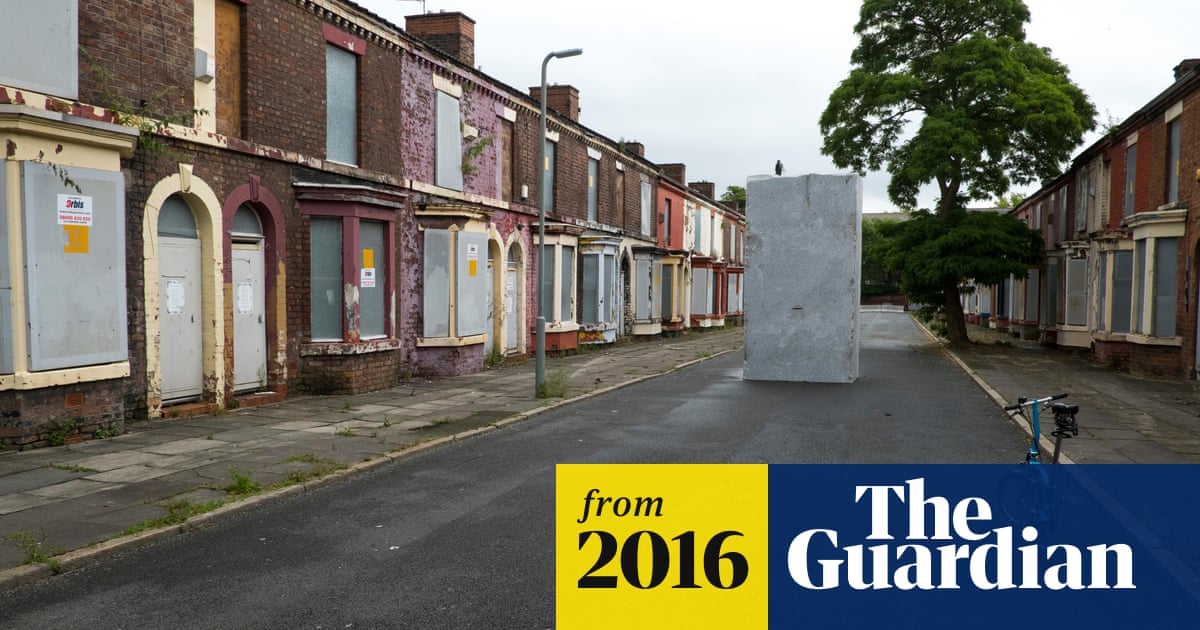The 2016 photograph, featured in The Guardian, depicts a desolate neighborhood street devoid of people and vehicles. The scene is characterized by a series of uniformly two-story, log-structure buildings flanking both sides of the road. These structures, presenting various shades of brown and yellow hues, are all boarded up, with doors and windows sealed shut. The sky overhead is a dull, overcast grey, contributing to the bleak atmosphere. In the middle of the street stands a large, enigmatic white concrete block or pod, drawing the eye as the central focal point. The street itself is barren except for a single light pole, a lone bicycle in the right-hand corner, and a tree in the background. The image, which features prominently displayed yellow and black text indicating "From 2016" and a blue background with white text reading "The Guardian," exudes an eerie silence and abandonment.